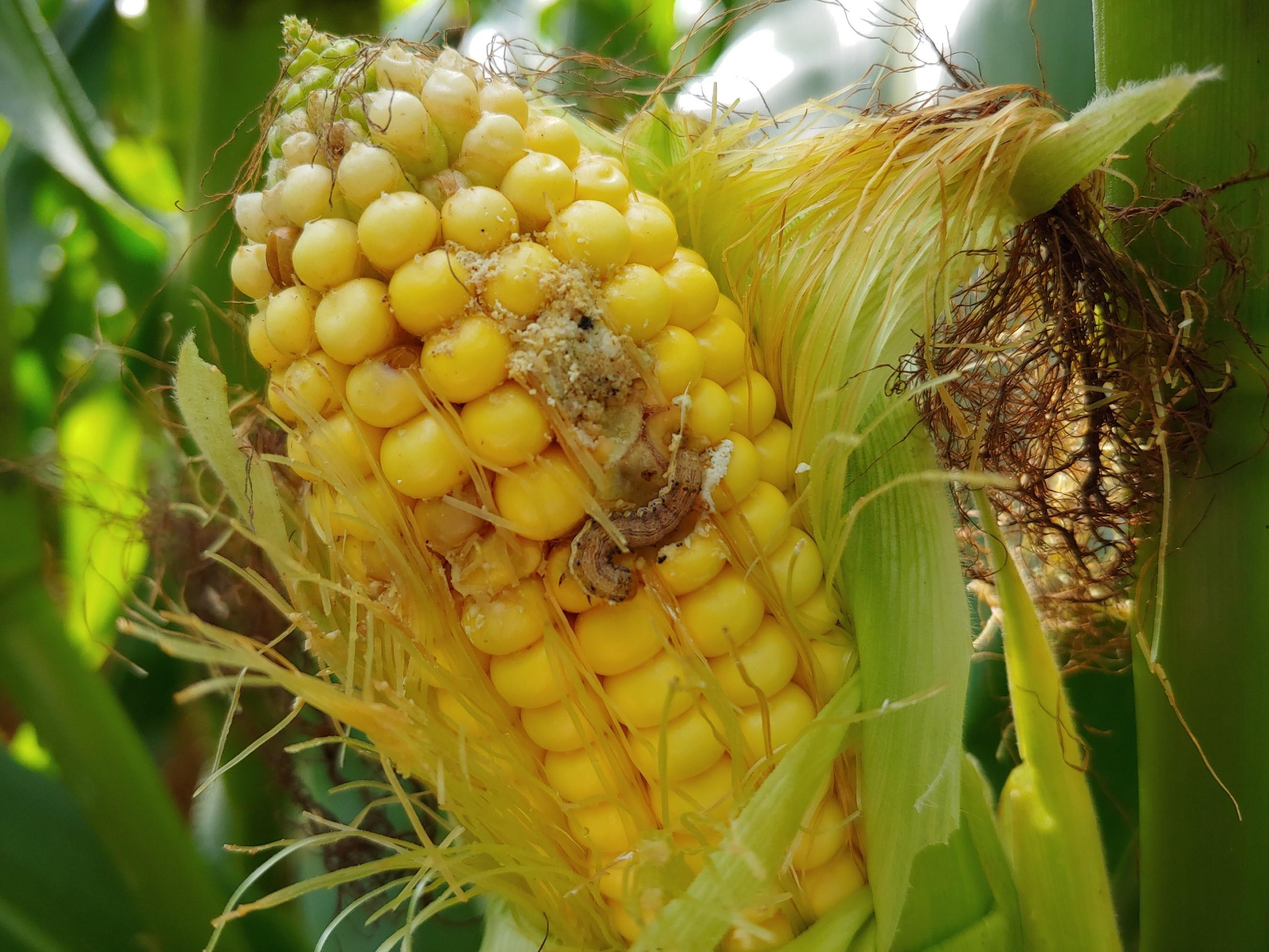This outdoor photo, set in a cornfield, shows a close-up view of an ear of corn still attached to the stalk. The green husk is slightly peeled back to reveal a mix of yellow and undeveloped green kernels. The silk fibers, some of which are brown and shriveled, hang loosely down the sides. Prominently featured is a light brown caterpillar or worm, about the size of a few kernels, situated halfway down the cob. It appears to be feeding on or nesting in the corn, creating visible damage to the kernels around it. The background is filled with large green leafy plants, with sunlight filtering through foliage, emphasizing the corn and its tiny invader.